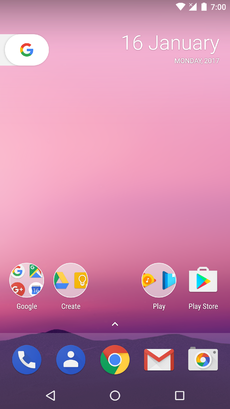The screenshot is taken from an Android device, capturing a moment at exactly 7 o'clock on Monday, January 16th, 2017. The device shows a full battery life and a strong Wi-Fi signal. The date and time are prominently displayed. The background of the screen features gradients of pink and purple.

On the left side of the screen, the iconic Google 'G' logo is visible, showcased in its familiar red, orange, green, and blue colors, set against a white oval background. Several Google applications are organized into different categories such as 'Google Maps,' 'Create,' 'Play,' and 'Play Store,' with the Play Store icon represented by a white briefcase adorned with a multicolored triangle.

At the bottom of the screen, several essential app icons are lined up: the 'Call' button, 'Contacts,' 'Google,' 'Mail,' and 'Camera.' Each icon is easily identifiable and neatly arranged, contributing to the organized and user-friendly interface of the device.